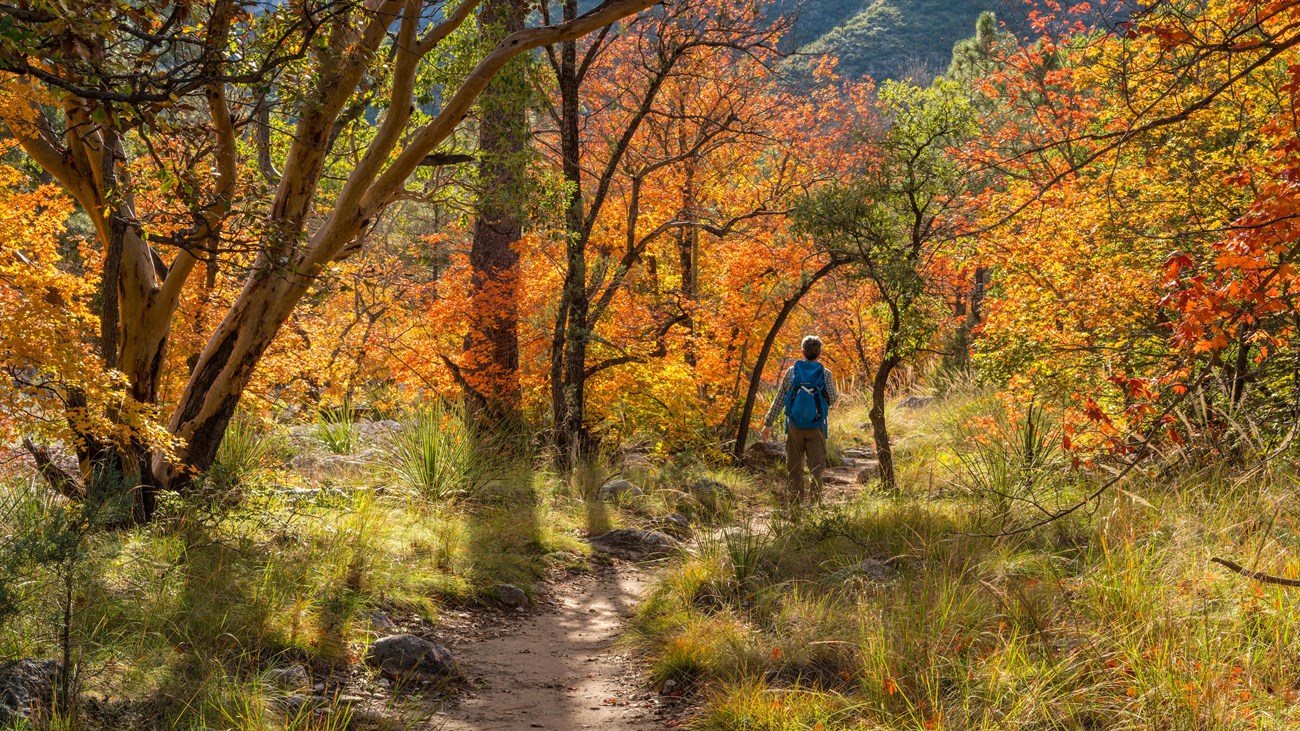This photograph captures a serene autumnal scene of a young man hiking on a narrow, brown dirt path through a picturesque forest. The man, whose back is to the camera, is adorned in khaki pants, a plaid shirt, and a blue backpack. The path begins at the bottom-center of the frame, meandering upwards before curving to the right, where it eventually disappears into tall grass. The ground on either side of the path is a vibrant green, despite patches of yellowish grass and areas shaded by the forest canopy. The trees, adorned in a mix of green, yellow, and orange leaves, hint at the transitional beauty of fall. In the background, well-forested mountains peek through the tree line, adding a majestic touch to this tranquil nature scene. The sunlight filters through the foliage in patches, casting a dappled light on the forest floor, creating a dynamic interplay of light and shadow.